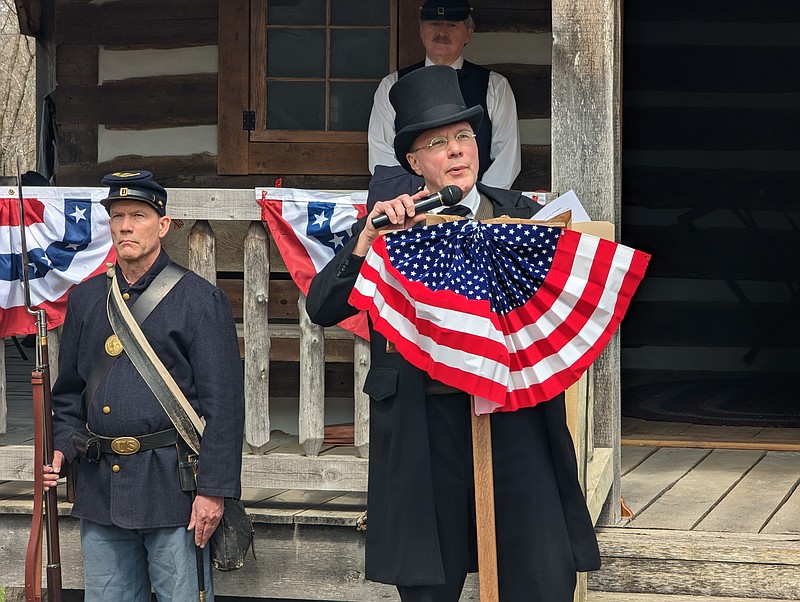In this color photo, a man dressed in a black top hat and long black coat stands at a slender wooden podium adorned with a folded, pleated American flag in a red, white, and blue pattern, resembling a half-circle. The man is mid-speech, holding a black microphone in his left hand. He wears glasses and stands on a wooden deck, likely part of a log cabin porch. To his left, a serious-looking man in a blue Civil War Union uniform, complete with a cap and an old-fashioned bayonet, stands watchfully. In the background, another man dressed in a white button-up shirt with a black vest and mustache observes the scene, adding to the historical ambiance. More red, white, and blue decorations can be seen on the porch railing, enhancing the patriotic theme of the setting.